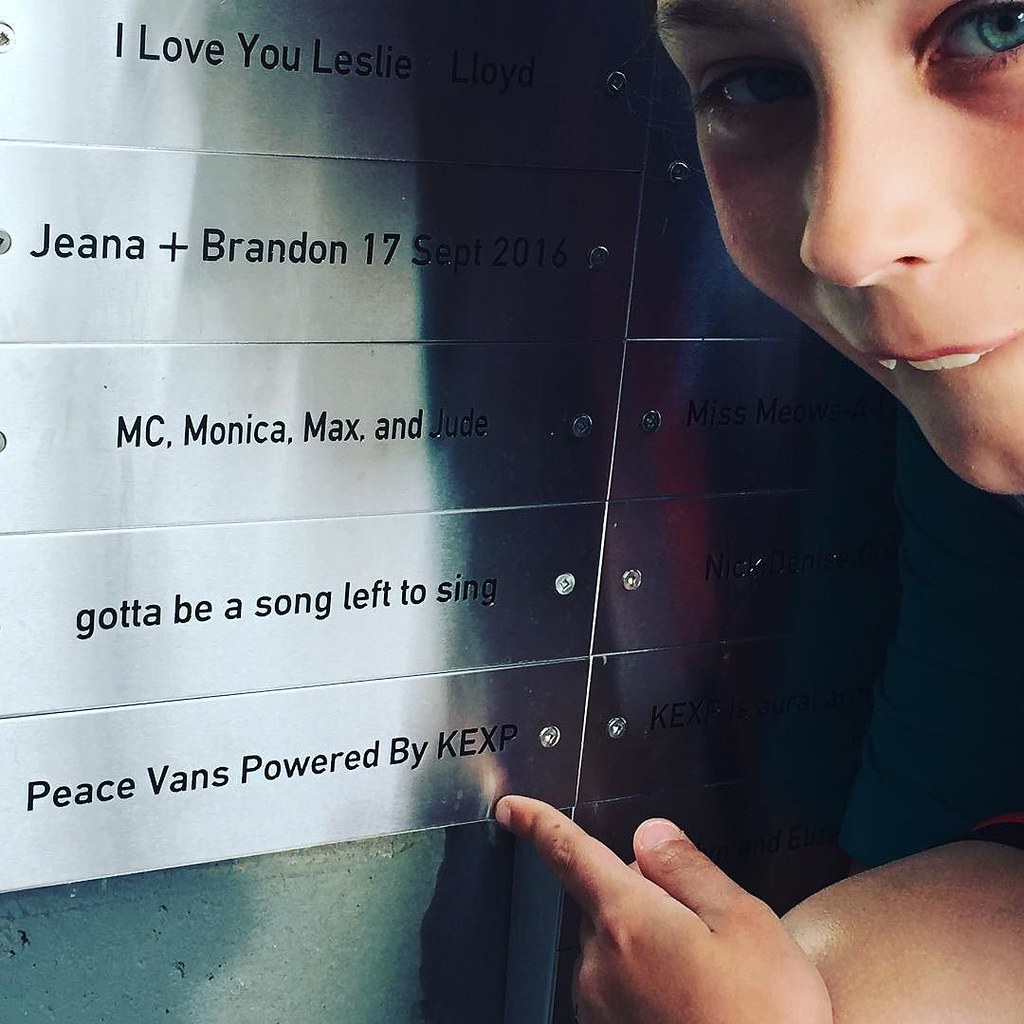A smiling adolescent, possibly male or female, is pointing at a series of etched stainless steel plaques mounted on a concrete or light green stone wall. The top left corner of the image features their white face, one blue eye partly shaded, captured by the light coming from the right. The person's hand, located in the bottom right corner, points specifically to the plaque reading, "Peace Vans powered by KEXP," attached firmly with screws or rivets. Above this, another plaque reads, "Gotta be a song left to sing," followed by "MC, Monica, Max, and Judy." Higher up, amidst a dark shadow with streaks of red and blue, is "Gina + Brandon, 17th of September, 1917" alongside other unreadable names obscured by the dim light. The multicolored shadow casts across the display, adding depth and texture to the structured arrangement of the etched names.